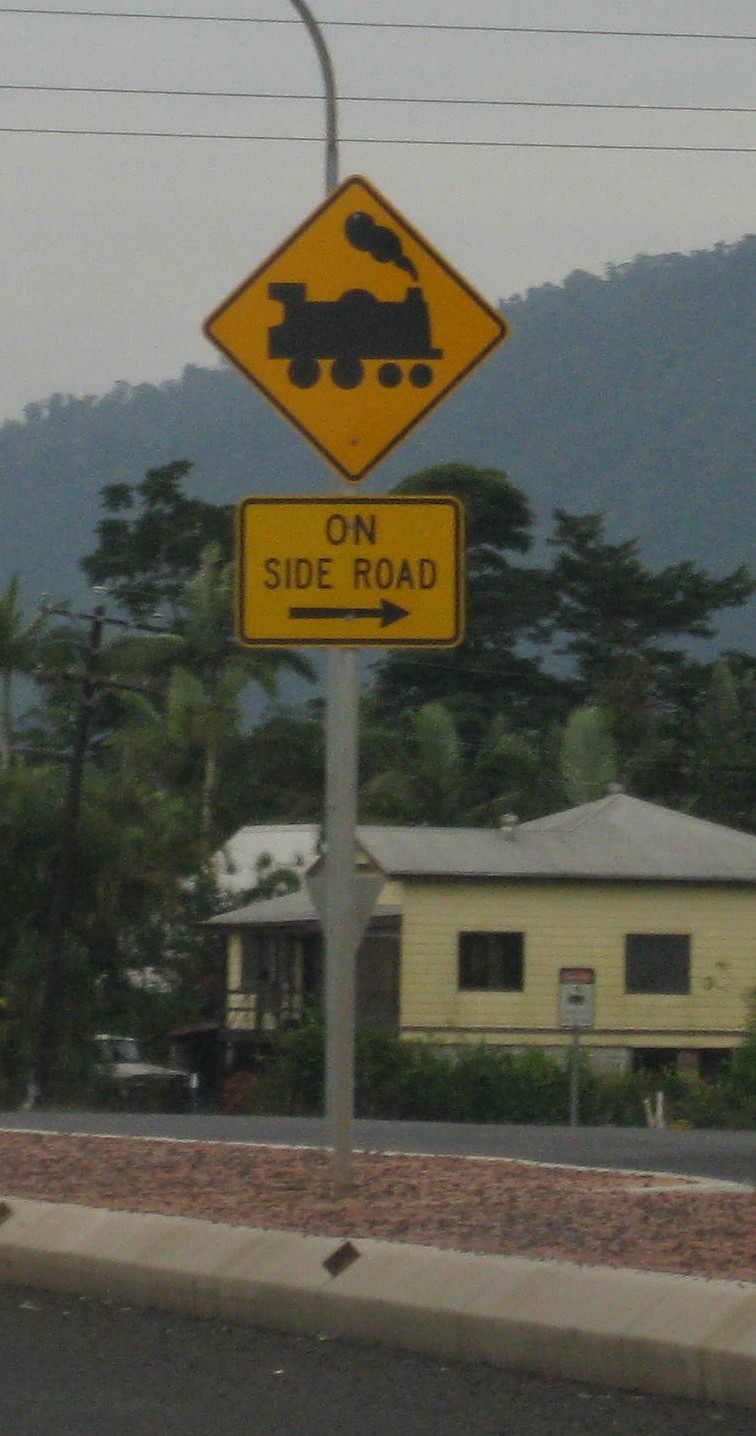The image depicts two road signs mounted on a single, medium-gray metal pole. The lower sign is rectangular and yellow with a black border, bearing the inscription "Side Road" accompanied by a black arrow pointing to the right. Directly above it, a triangular yellow sign with a black border portrays the silhouette of a train engine, complete with four wheels, a smokestack, and illustrated smoke emanating from the front of the smokestack.

In the background, there is a light-colored house, possibly painted yellow or cream, with a gray roof. Partially obscured by the pole and signs, there is another sign in red and white, though its text is unreadable. The signs are positioned on an island curb line, featuring two adjacent curbs separated by a reddish patch of dirt. Beyond the house, the scene includes lush trees and a very gray sky, with what appears to be the base of a mountain or hillside visible among the greenery.